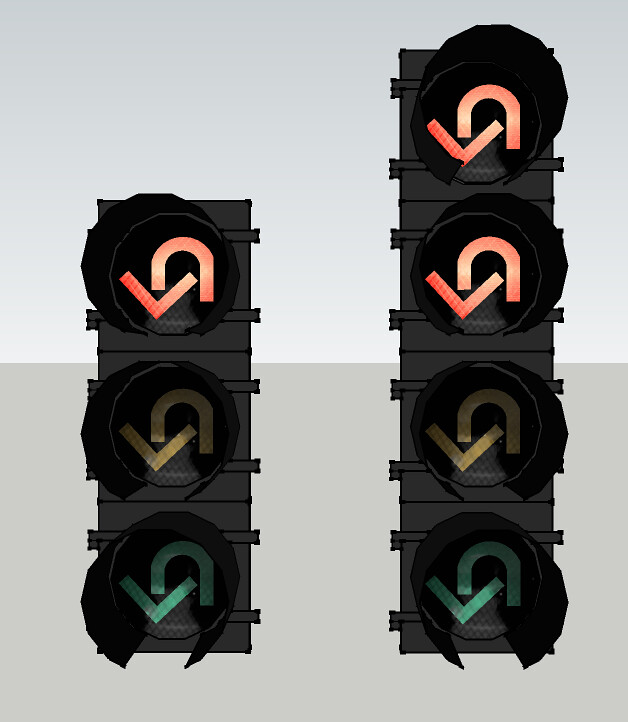This image is a detailed illustration of two artistic traffic signals set against a color-blocked background. The background consists of a medium gray rectangle at the bottom and a pale gray rectangle at the top. Each traffic signal features U-turn arrows instead of standard circular lenses. The signal on the left has three lenses: a red lens at the top, a yellow lens in the center, and a green lens at the bottom. The signal on the right has four lenses: two red lenses at the top, followed by a yellow lens, and a green lens at the bottom. The arrows on all lenses create a tunnel-like arch, making a U-turn shape. In this illustration, the red lenses on both traffic signals are illuminated.